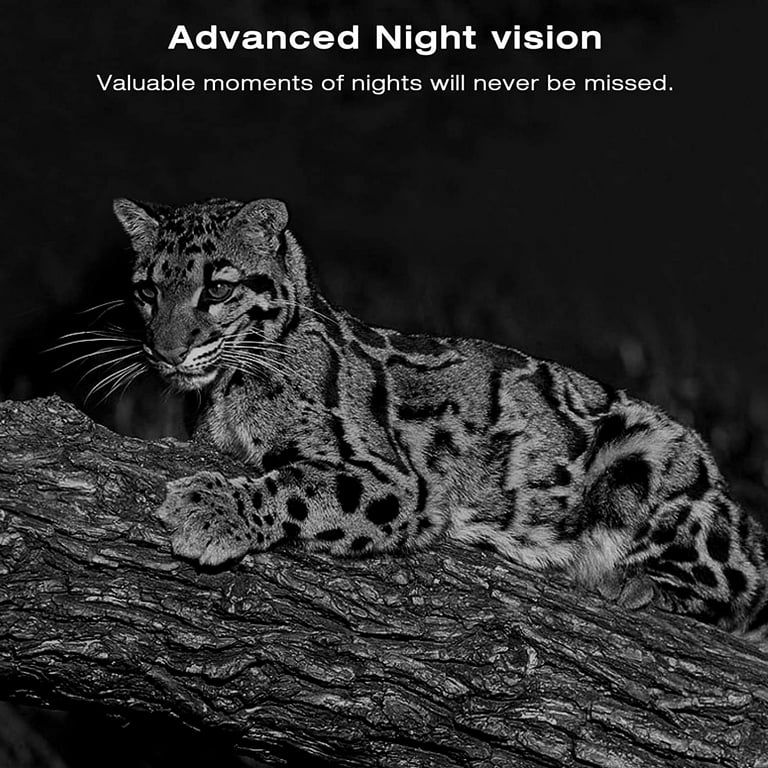This black-and-white photograph, likely an advertisement, features an evocative nighttime scene highlighting the advanced capabilities of night vision technology. At the top of the image, white text reads, "Advanced Night Vision," with "Valuable Moments of Nights Will Never Be Missed" written just below. Dominating the bottom half of the photograph is a thick tree log, upon which a poised young leopard sits. The background is deeply blurred and almost entirely black, accentuating the leopard's vigilant stance. The leopard faces left, its large eyes and ears alert as if hunting or observing something in the distance. Detailed patterns and stripes are distinctly visible despite the monochromatic palette, emphasizing its sleek form against the shadowy backdrop. Long whiskers extend from the leopard's muzzle, which, combined with its crouched posture, conveys a profound sense of nocturnal readiness.